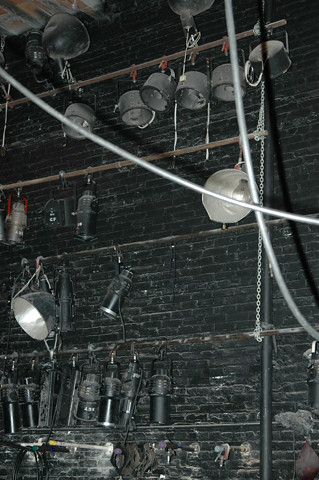This indoor color photograph taken in low light captures a complex stage lighting setup against a black painted brick wall, which appears somewhat dusty. The scene features a partially visible pipe rack extending vertically and occupying most of the image, with several gaps in the far right and top sections. Four horizontal pipes support an array of stage lights in various configurations and types.

Starting from the bottom, the first pipe holds a dense collection of long, skinny black cylindrical stage lights, primarily concentrated towards the middle left section. The second pipe above it is more sparse, holding a variety of lights including five to seven rectangular black cylinders and a large circular light with a silver center. Further up, the third pipe supports a mix of skinny and short, fatter cylindrical lights, with three easily visible on the left side—a large silvery circular light, a skinnier one, and another slightly shorter but still cylindrical one. The final top pipe features an assortment of lights similar in shape, mostly short cylinders with large bulbs.

Two silver cables are stretched diagonally across the image: one descending from the top and exiting to the right, and another originating from the left corner and also heading towards the right in an X pattern. The entire setup lacks any text or printing, focusing purely on the technical complexity of stage lighting equipment.